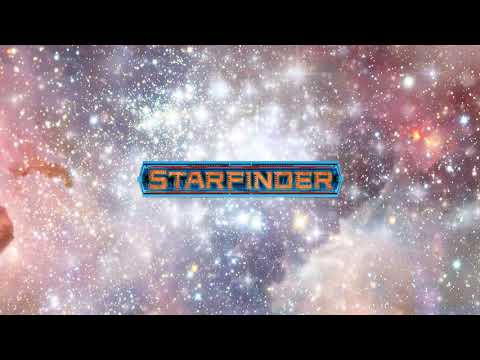The image is a colorful and vibrant cover art, possibly the title image of a game called "Starfinder." The background depicts a starlit sky, reminiscent of a galaxy or nebula, with stunning hues of deep purple, soft pinks, oranges, and rose colors all blending seamlessly. Glittery, sparkly clouds spread across the scene, with clusters of white stars varying in size, adding a striking celestial effect. Centrally positioned is a prominent blue text box or plaque, featuring the word "Starfinder" in all capital letters. The lettering is in a bold orange or gold color, standing out clearly against the cosmic backdrop. The design is both eye-catching and immersive, highlighting the game's space theme effectively.